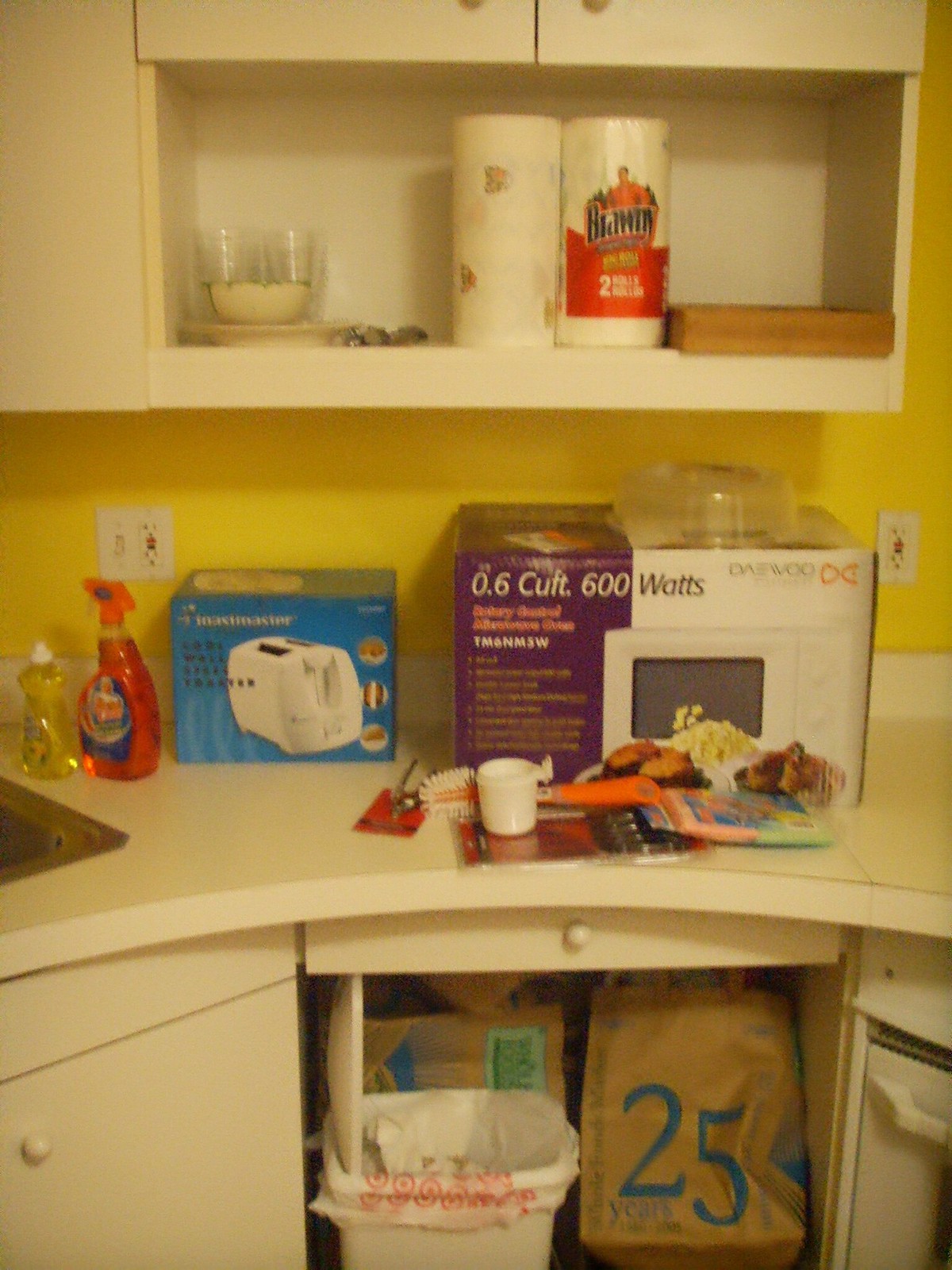This photograph captures a detailed view of a home kitchen. The image showcases a segment of the kitchen, highlighting the upper cabinets, counters, backsplash, and lower cabinetry.

The upper cabinets are white, and partially in view are two doorknobs at the top of the image. Beneath these doors is an open shelf displaying a brown wooden box on the right, alongside two rolls of paper towels, with the roll on the right prominently featuring the Brawny logo. On the left side of the shelf, there are several white bowls, a white plate, and a collection of clear glass or plastic cups in the background.

The backsplash of the kitchen is painted a lively yellow, broken up by two visible electrical outlets. To the far left, the corner of a metal sink is just visible, signaling the edge of the counter space. On the countertop, there is a bottle of yellow dish soap and an orange Mr. Clean cleaning product. Next to these, a blue box featuring an image of a white toaster sits on the counter. Another box on the right side, colored purple and white, depicts a white microwave with specifications indicating it has 0.6 cubic feet and 600 watts of power.

The white countertop itself is curved, and various other kitchen items are scattered around. Below the counter is a thin drawer, directly above an open lower cabinet. Inside this cabinet, paper bags and a white trash can lined with a Target bag are visible. The photograph provides a comprehensive look at one portion of this homey and functional kitchen space.